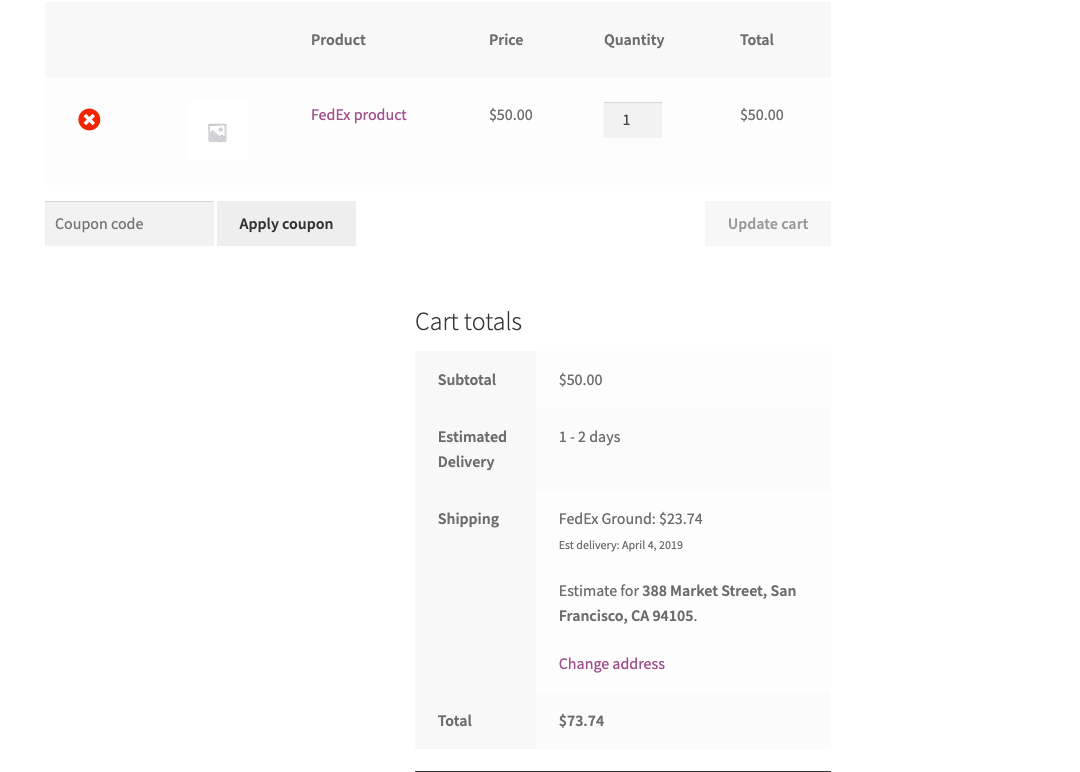This is a screenshot of an e-commerce website's final checkout page, detailing the total amount due, along with product and pricing information. At the top, there is a neatly organized chart featuring columns labeled “Product,” “Price,” “Quantity,” and “Total.” 

- Under "Product," a single item is listed: "FedEx service."
- The "Price" column shows "$50."
- The "Quantity" column indicates "1."
- The "Total" column confirms the total price as "$50."

To the left of the listed "FedEx service," there is a red "x" icon, presumably for removing the item from the cart.

Below the product details, on the bottom left of the chart, there is a coupon input area with a text bar for entering a code and an "Apply Coupon" button beside it. Adjacent to this, on the bottom right, there's an "Update Cart" button for revising the cart contents.

Towards the bottom right section of the page, a section titled “Cart Totals” provides a summary:

- "Subtotal" is listed as "$50."
- "Shipping" showcases "FedEx Ground" priced at "$23.74."
- "Estimated Delivery" is indicated as "1-2 days" with an expected delivery date of "April 4, 2019."
- The complete address "San Francisco, CA 94105" is also shown with a "Change Address" option.
- The final "Total" is calculated as "$73.74."

All these elements are displayed on a clean, white background.